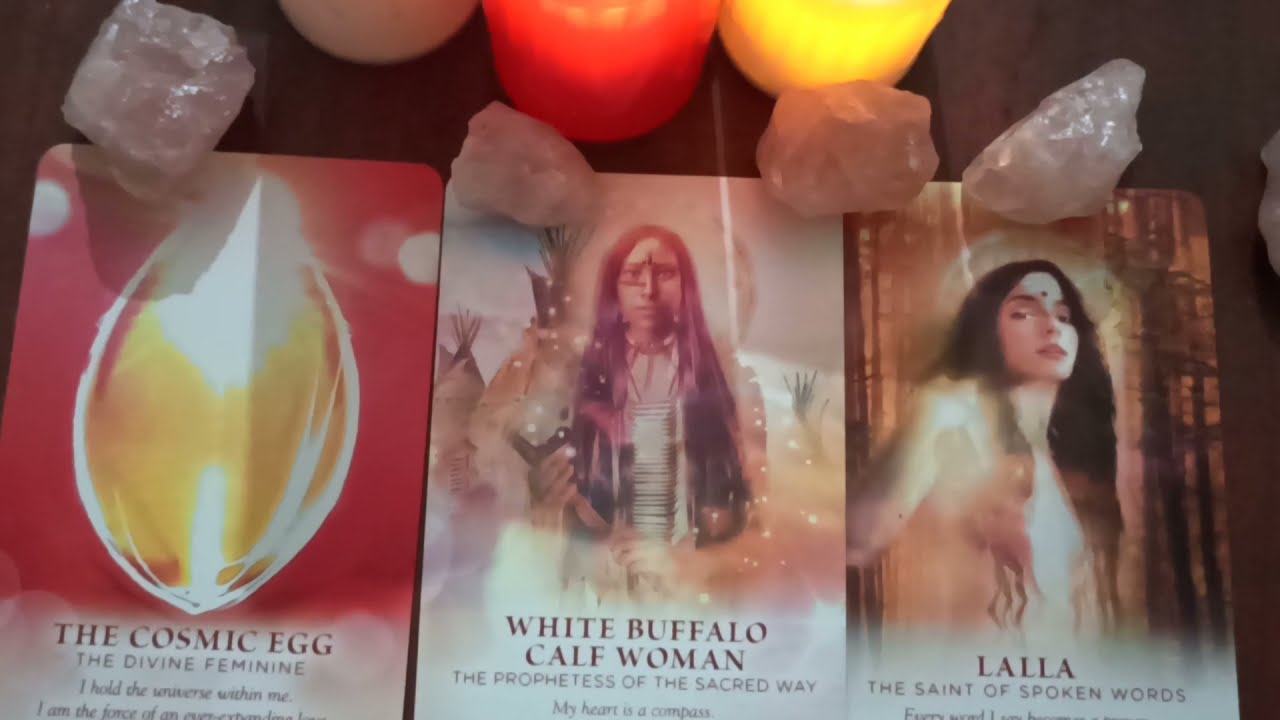The image displays a set of three spiritual or tarot-like cards laid out on a dark brown wooden table, partially adorned with crystals and candles. The card on the left, predominantly red with an illustration of a yellow, luminescent spherical shape resembling a cosmic egg, is titled "The Cosmic Egg, The Divine Feminine." The text beneath it reads, "I hold the universe within me, I am the force of..." but the rest is cut off by the bottom of the frame. The middle card features "White Buffalo Calf Woman, The Prophetess of the Sacred Way," depicting a Native American woman with black hair, center-parted, dressed in traditional garb, and holding a tool. The background subtly shows three teepees. The card on the right is labeled "Lalla, The Saint of Spoken Words," and portrays a woman with long black hair and a dot on her forehead, possibly unclothed, with a background of indistinct brown pillars or streetlights. Suspended above the cards are objects likely to be quartz crystals and three lit candles; a red candle in the center, a mostly cropped yellow candle to the right, and a partially visible white candle to the left. The scene captures a mystical, contemplative atmosphere.